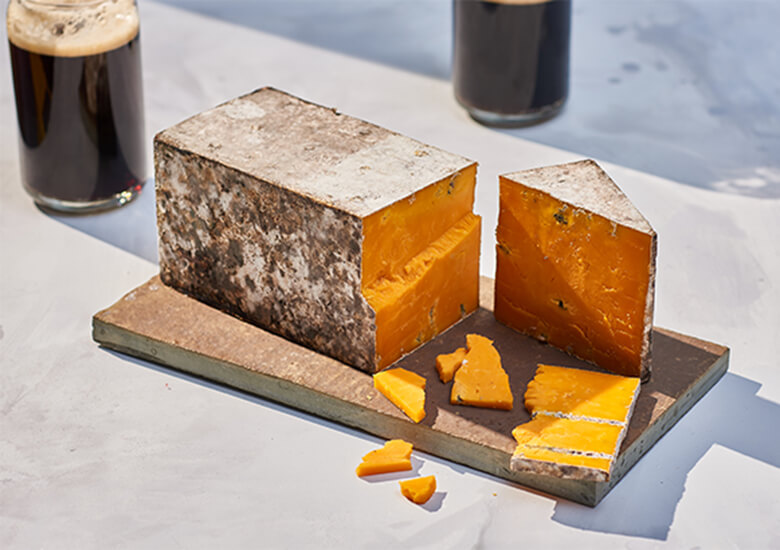The photograph features a rectangular block of cheese, prominently placed on a wooden cutting board resting on a smooth, white surface. The cheese appears to be quite old or aged, with a brownish and white, moldy-looking crust. The inner part of the cheese is vividly bright orange, resembling an artificially colored cheddar. The block has been partially sliced, revealing a mix of smooth cuts and broken, crumbly edges, with several pieces scattered around the cutting board. The scene is illuminated by light that casts distinct shadows of the cheese and two glasses of a frothy, dark drink—possibly Guinness stout—positioned behind the cheese.